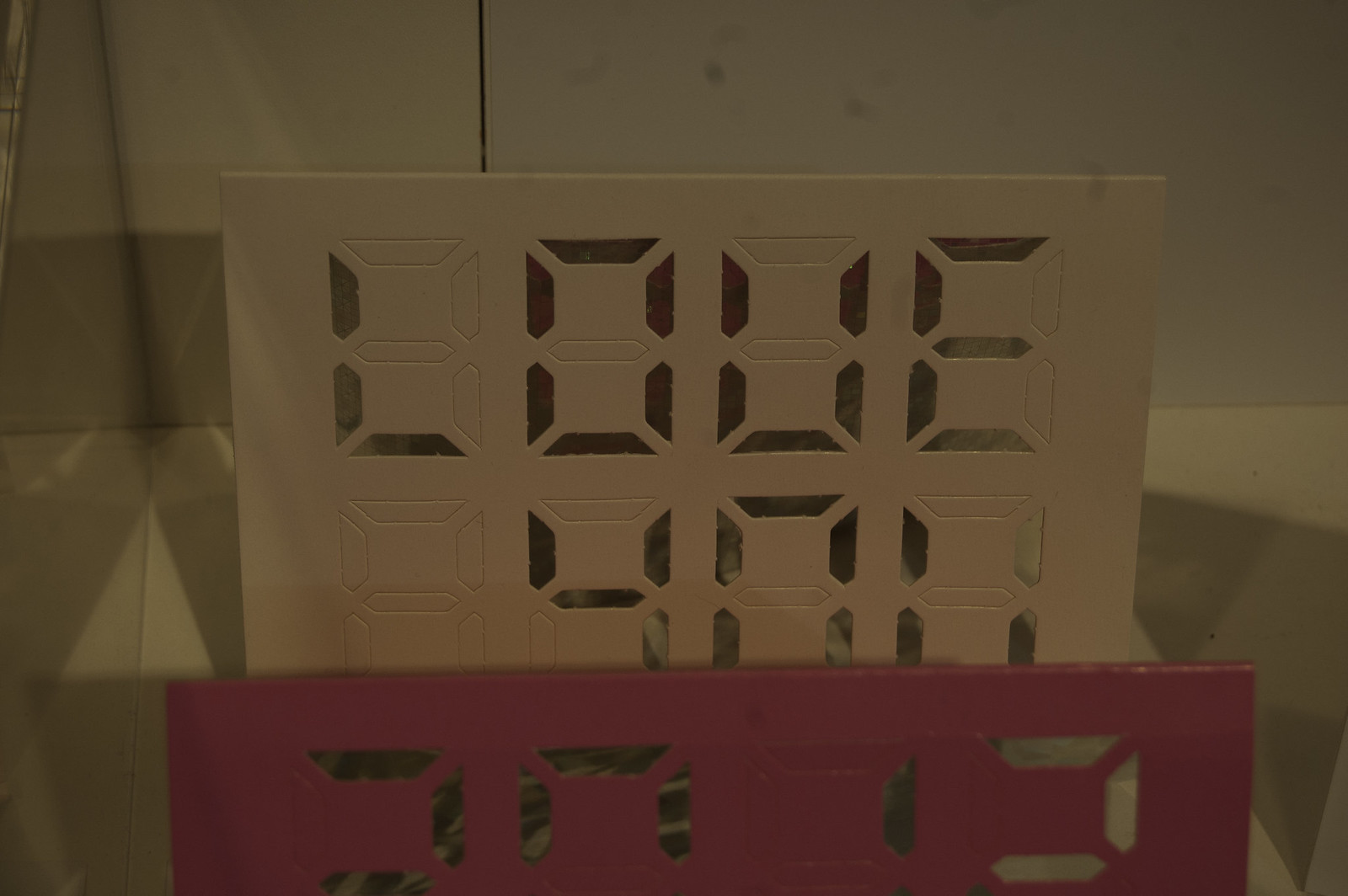This photograph captures a customizable item made from thin sheets of metal, designed to allow for personalized messages. There are two square metal pieces featured; one is a subtle cream or white, while the other is a bold red. Both pieces are perforated with small dashes arranged in the shape of figure eights, offering a grid that can be selectively punched out to form letters and numbers. The white metal piece has been carefully punched out to reveal a heartfelt message. The top row spells out "LOVE," and the bottom line reads "YOU," making it a unique and sentimental keepsake.